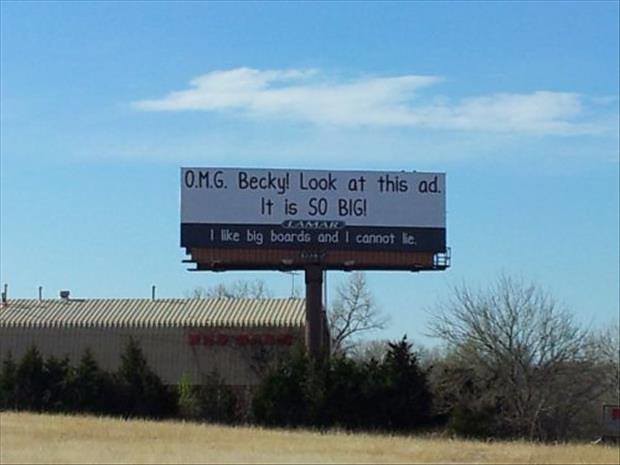This is an image featuring a large billboard set against a scenic backdrop. The billboard displays bold text, reading: "Oh, I'm Jerry M.G. Becky!" followed by an emphatic exclamation point. Both the size and design of the advertisement make it stand out prominently. The advertisement includes a playful tagline at the bottom, "I like big boards and I cannot lie," which references a popular song lyric. The text is encapsulated by a green border.

The billboard is mounted on a thick brown pole and includes a small walkway at its base, suggesting maintenance access. It is likely positioned alongside a highway, making it visible to passing drivers. In the surrounding area, there are a mix of evergreen trees and leafless trees, indicating that the season might be late fall or winter. Additionally, there's a warehouse nearby with red lettering that is not fully legible in the photograph. The overall scene combines industrial elements with a touch of nature.